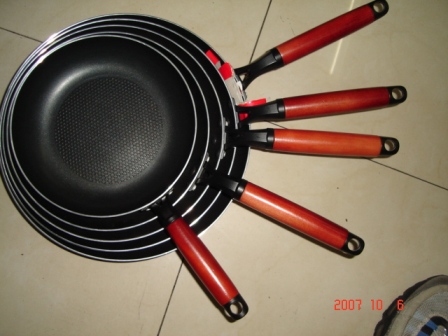This photograph, taken on October 6, 2007, depicts a set of five black Teflon pans arranged on a tiled kitchen floor. Each pan features a matching red handle with a loop at the end, allowing them to be hung. The pans are stacked according to size, with the largest at the bottom and the smallest at the top, and their handles fan out without overlapping. The kitchen setting is indicated by the visible floor tiles and a glimpse of the photographer's shoe—a white sneaker with blue trim—in the bottom right corner. The lighting from above highlights the shiny surfaces of the pans and the neat arrangement.